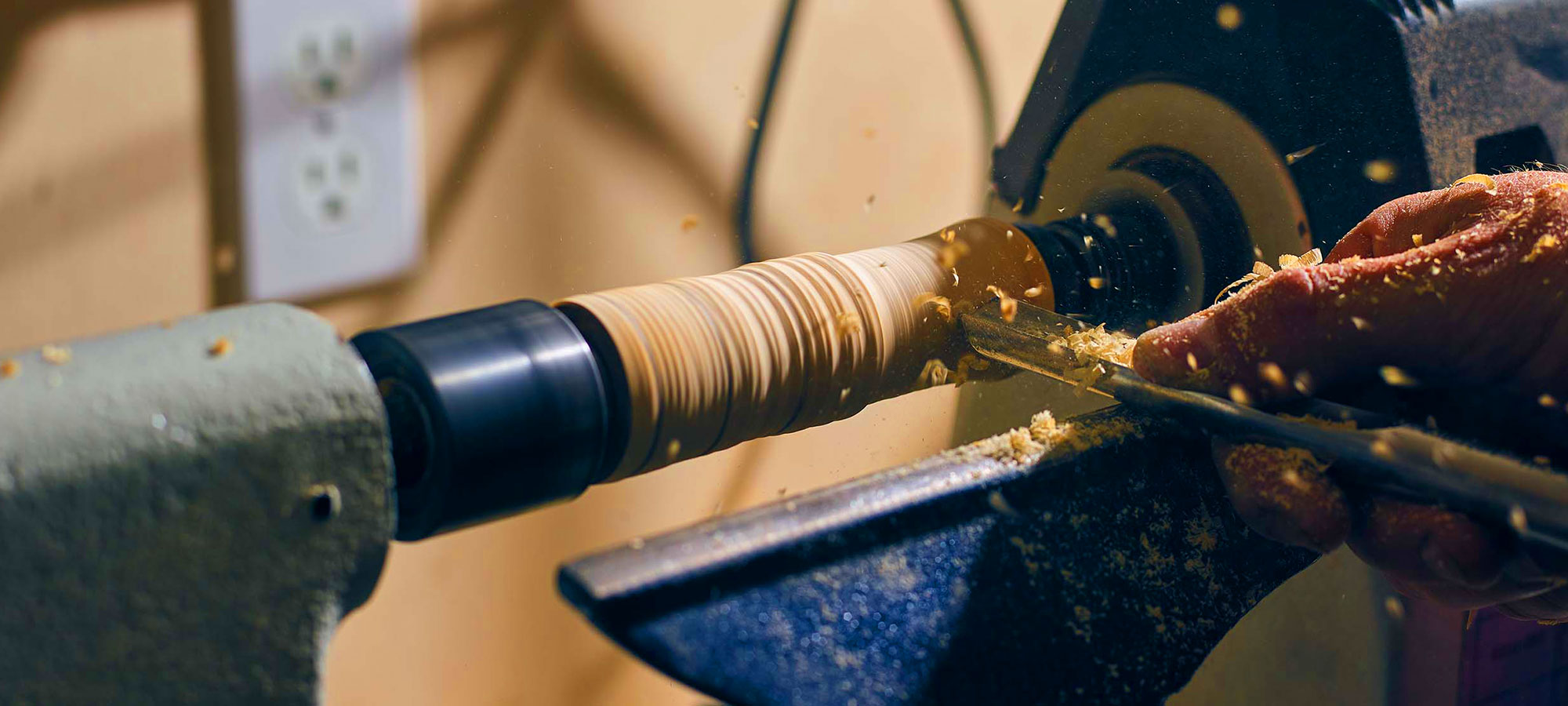The image depicts a wooden lathe in action, capturing a detailed scene of woodturning. At the center of the scene, a light tan cylindrical piece of wood is clamped between two blue metallic clamps – a larger one on the right and a smaller one on the left. The wood is spinning rapidly as a person's hand, visible on the right, carves into it with a sharp, gray metal tool. Wood shavings and chips fly off in various directions, and the person's hand is covered in sawdust. The lathe's base features a significant metal structure with a wheel, and in the foreground, a blue blade-like leveler, or brace, supports the carving tool. The background is softly out of focus, showcasing a cream-colored wall with an electrical outlet. The spinning wood, likely being shaped into a table leg, exhibits numerous grooves from the ongoing carving process.